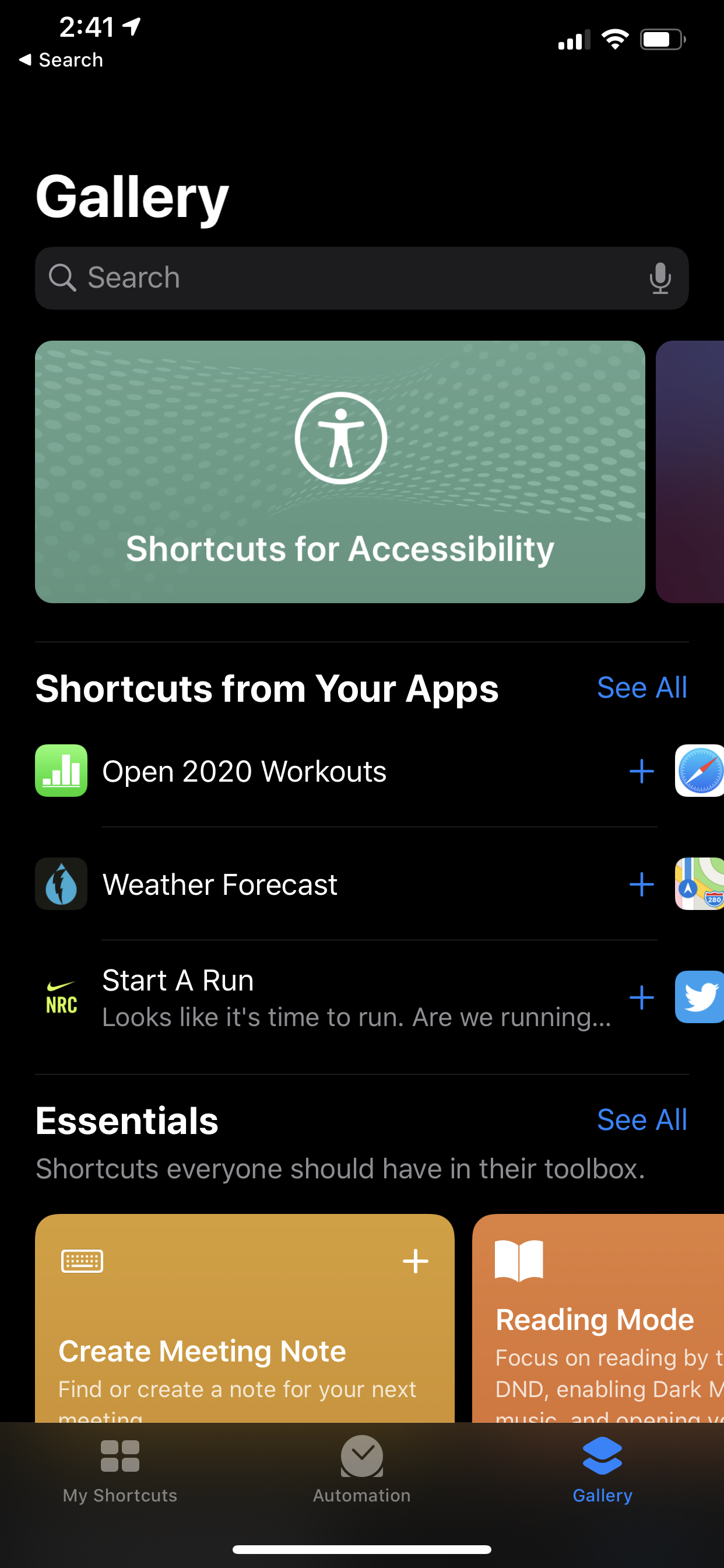This is a detailed screenshot of a cell phone screen. In the upper left corner of the screen, the time is displayed as 2:41, though it is unclear if this is AM or PM. To the right of the time, there is a Telegram icon, which resembles the insignia from Star Trek uniforms. At the very top right, the screen shows a battery indicator that is nearly full, a Wi-Fi indicator with three out of four bars, and a cellular signal indicator also with three out of four bars.

Just below these indicators, on the left side, there is the word "Gallery" in white letters. Below that, there is a search bar with a magnifying glass icon on the left and a microphone icon on the right side. Underneath the search bar is a large blue-green rectangle with white text that reads "Shortcuts for accessibility." Within this rectangle, there is a white circle featuring a simplistic person figure, also in white. Adjacent to this blue-green rectangle, but partially cut off on the right side of the screenshot, is a blue and purple rectangle.

Further down, the text "Shortcuts from your apps" is written, followed by a blue hyperlink on the right that says "See all." Below this, there are several options listed: "Open 2020 Workouts," "Weather Forecast," and "Start a Run." The caption concludes with "It looks like it's time to run. Are we running..." indicating a prompt or question related to starting a run.